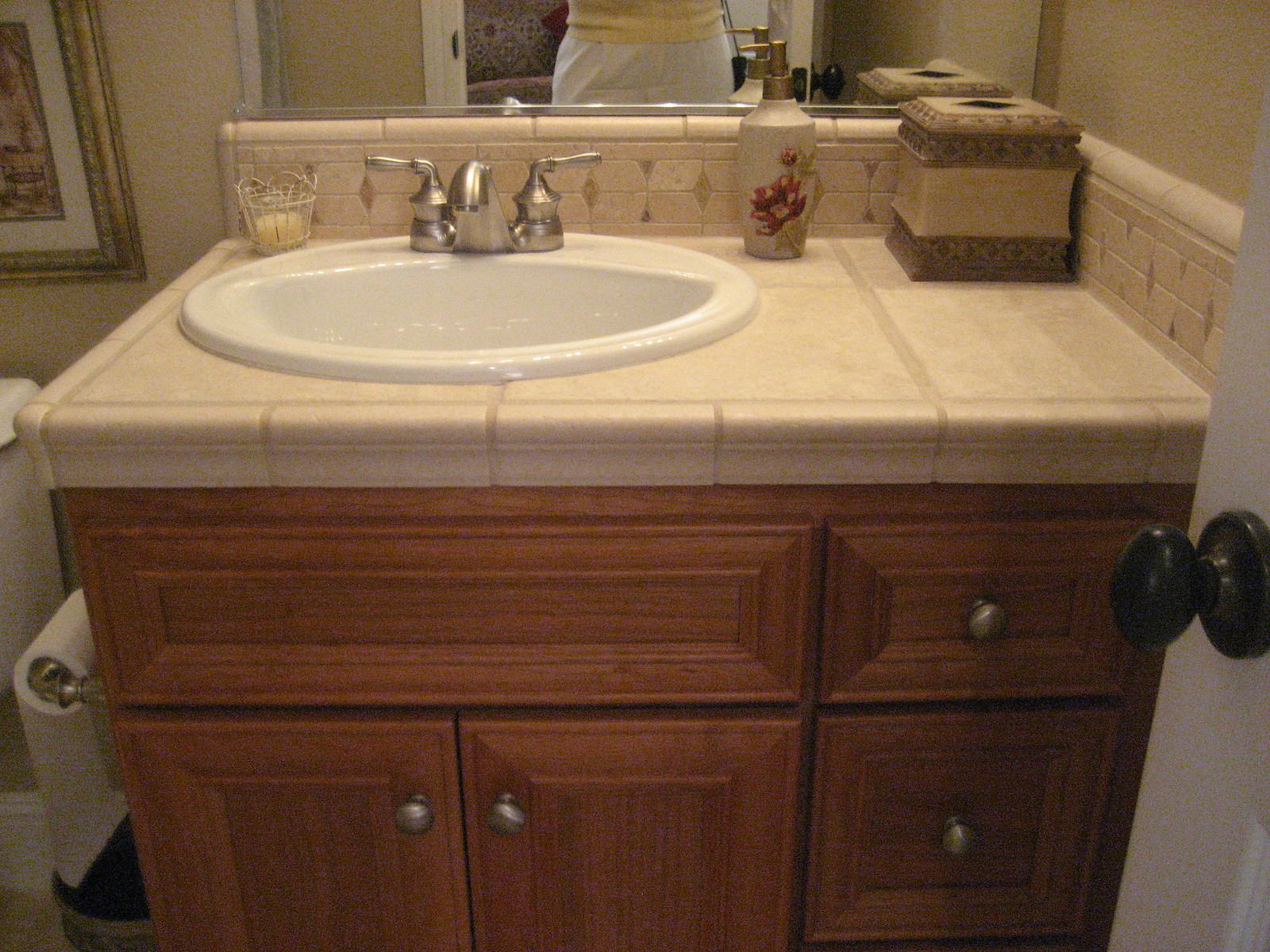In this photograph of a small bathroom, presumably not the master bathroom, the focus is on a tiled countertop adorned with a decorative soap dispenser, a stylish tissue holder, and a delicate candle arranged towards the left of a white porcelain sink. The sink features a modest spout and contemporary brushed nickel fixtures. To the left of the sink cabinet, which is crafted from wood with a light red tone, there is a toilet paper holder. The cabinet handles match the brushed nickel of the sink fixtures, although the door handle shows a black tarnished brass finish. The top part of the toilet tank is visible but partially cut off at the left edge of the frame. Above the toilet, a framed portrait hangs on the wall. Behind the toilet paper holder, an item that may be a brush or a plunger is faintly discernible. The person capturing the image is partially visible, showing only the lower part of their shirt and the top of their pants, which are yellow and white, respectively.